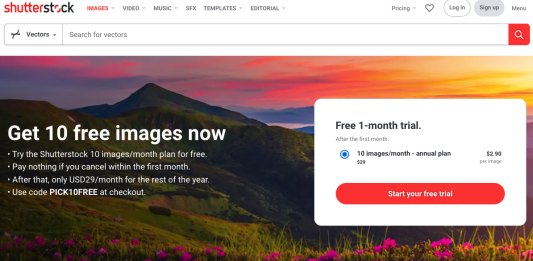The screenshot, captured in landscape mode and in color, showcases the Shutterstock website on a computer screen. Shutterstock, a popular platform for sourcing free images, has its distinctive red and black logo prominently displayed at the top. The navigation bar directly underneath the logo lists the available tabs: Images, Video, Music, SFX, Templates, and Editorial. Below the navigation bar is a "Search for Vectors" feature, enabling users to type in specific vectors and initiate a search.

Situated on the upper right of the interface are additional features: a Pricing link, a heart button for favoriting items, and a Log In/Sign Up menu. Dominating the center of the image is a prominent banner advertising a limited-time offer to "Get 10 Free Images Now." This banner is set against a scenic background depicting a picturesque mountain landscape adorned with wildflowers and lush green brush.

The promotional text on the banner informs users of a special deal: they can try Shutterstock's 10 images a month plan for free. The offer stipulates no initial payment if canceled within the first month, and a subsequent cost of USD $29 per month thereafter.